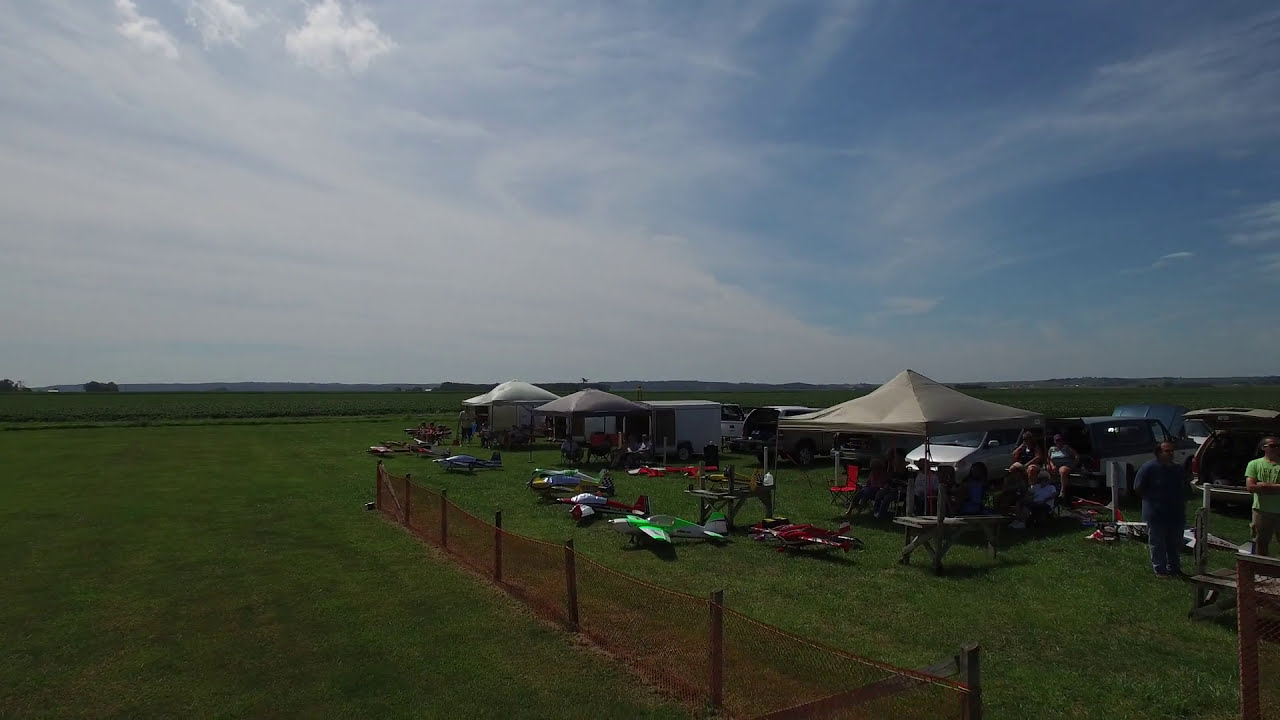This color landscape photograph, taken from a drone, captures a vibrant and casual outdoor event focused on miniature aircraft racing. The image is dominated by green grass and a blue sky, highlighted with thin, cirrus clouds. In the center and right of the photograph, various pop-up tents form a makeshift canopy under which numerous people are milling about. To the left, a row of small, remote-controlled model airplanes, some approximately three to four feet long, are lined up on the grass. The models are brightly colored, including distinct shades of green, blue, red, and tan, with one vivid green plane particularly standing out. The canopies, model planes, and scatter of participants create a lively atmosphere. A mesh fence stretches across the grassy field, supported by wooden posts, acting as a barrier. At the background, parked cars are visible, adding to the casual, recreational ambience. The photograph, casually snapped by an onlooker's drone, incidentally captures the extensive green fields in the distance with no text or significant professional staging evident. The overall setting conveys an informal gathering under natural lighting, emphasizing community and hobbyist energy in a realistic, representational style.